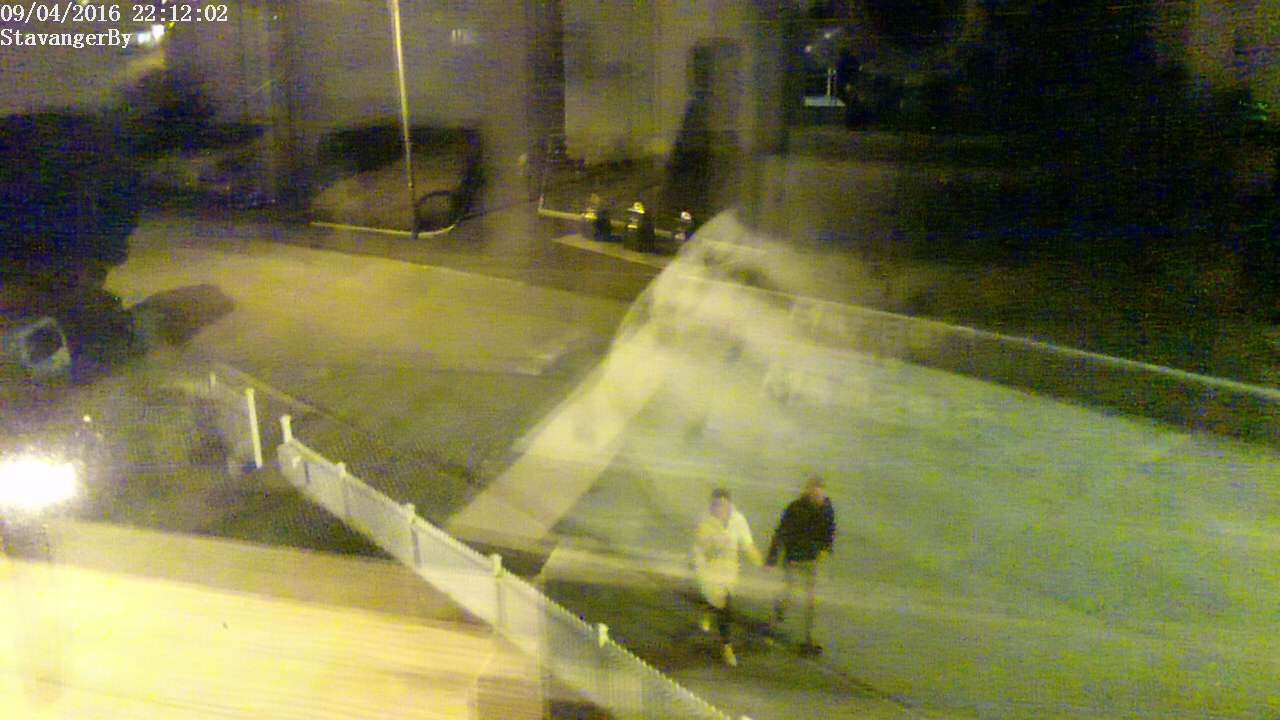This photograph, seemingly captured by a security camera, shows a couple walking hand-in-hand in an outdoor setting. The image is taken through glass, producing a slight blurry reflection that spans much of the frame. The couple is distinctly visible, with one person wearing a black top and the other in a white top, creating a striking contrast. They stroll alongside a classic white picket fence, adding a quaint touch to the scene. Surrounding them is an industrial area featuring parked cars and a building adjacent to a sidewalk. A timestamp in the lower corner of the image reads "09-04-2016," marking the date of this captured moment.